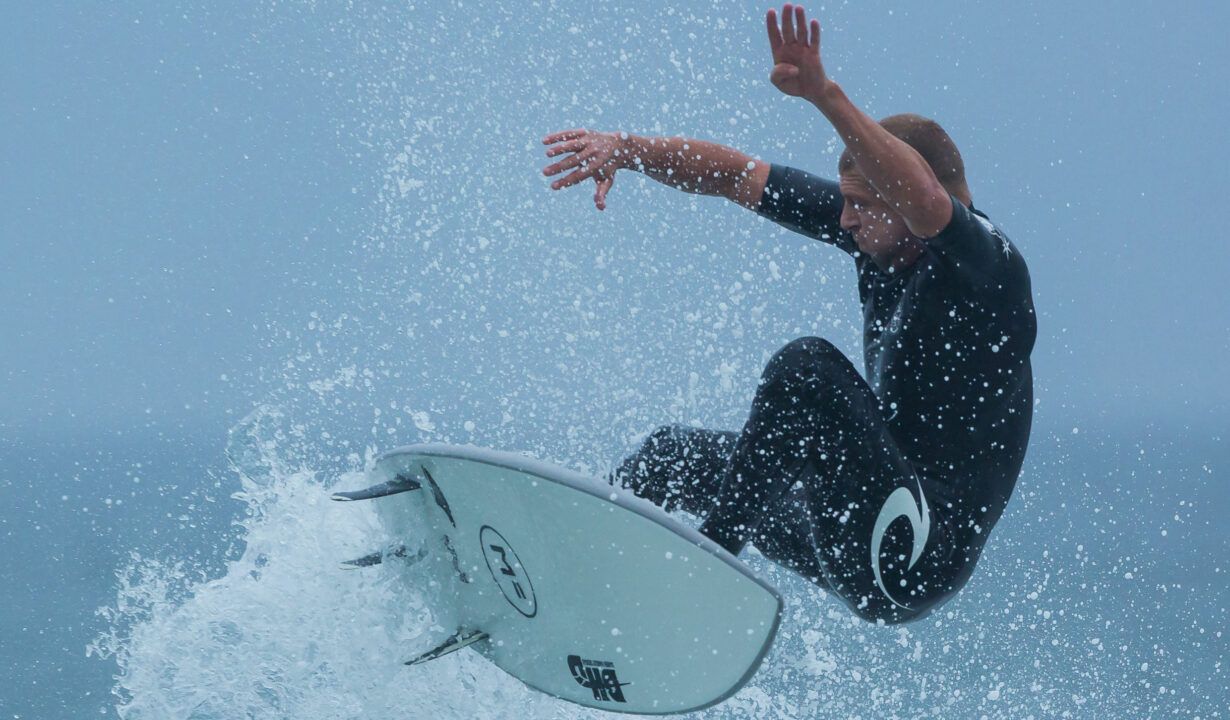The photograph captures an intense action shot of a surfer in mid-surf, expertly navigating a wave. He is airborne, with his arms spread wide to maintain balance as the surfboard, nearly vertical, reveals its aqua blue underside complete with three fins and brand logos. The surfer sports a sleek, black full-body wetsuit, accented by an aqua blue swirl on the thigh. The dynamic scene is set against a backdrop where the deep blue ocean meets the lighter blue sky, both halves blending seamlessly. The power of the ocean is emphasized by the splashing water and foamy white waves, framing the surfer dramatically. The image is sharply focused and professionally composed, capturing the surfer's short hair and every detail of his thrilling maneuver in vivid clarity.